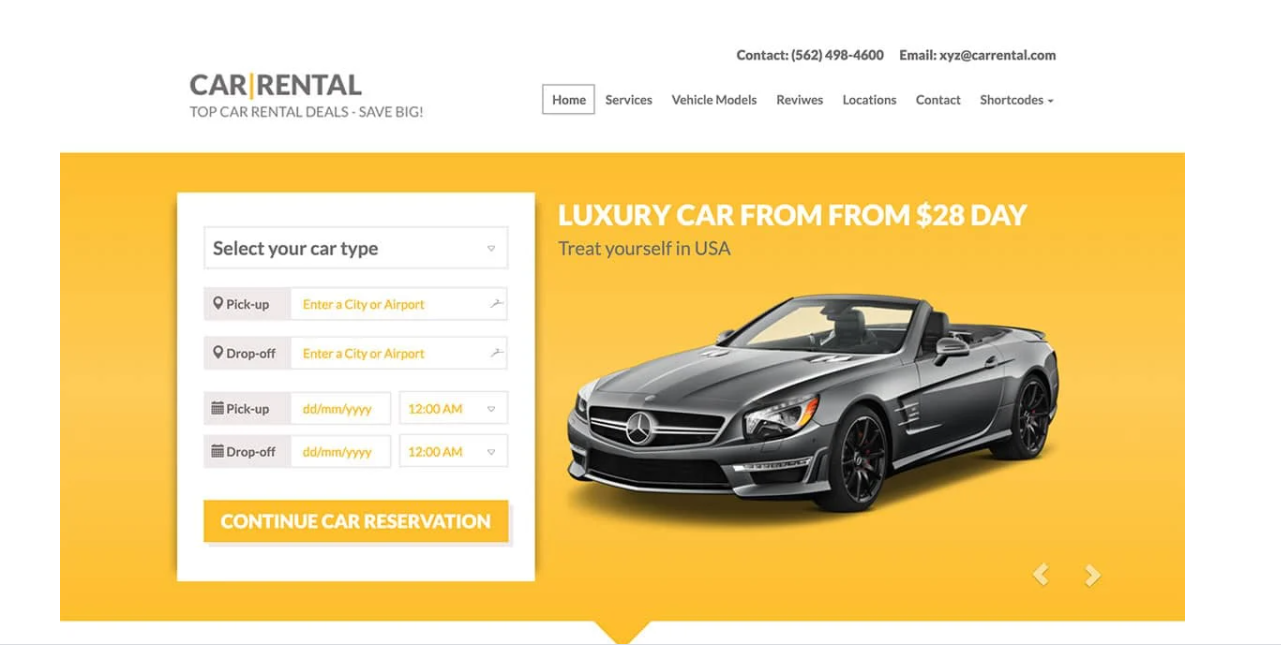The image is a screenshot of a car rental company's website predominantly featuring a vibrant yellow background. At the top left, in a bold white font, is the company logo "Car Rental," slightly larger than the accompanying text "Top car rental deals" and "Save Big." The top right displays contact details including a phone number and an email address. Below this, a navigation menu offers tabs for Home, Services, Vehicle Models, Reviews, Locations, Contact, and Shortcuts.

The central yellow area, which dominates the image, showcases a sleek pewter gray convertible, identified as a Mercedes. Adjacent to the car, the text announces, in capital letters, "Luxury Car from $28 a day," accompanied by the phrase "Treat Yourself in USA" in a distinctive gray font. To the left, a white square contains dropdown menus and fields for users to select car type, enter pickup and drop-off locations (city or airport), and specify date and time for both actions. Beneath these fields, a prominent yellow button prompts users to "Continue Car Reservation."